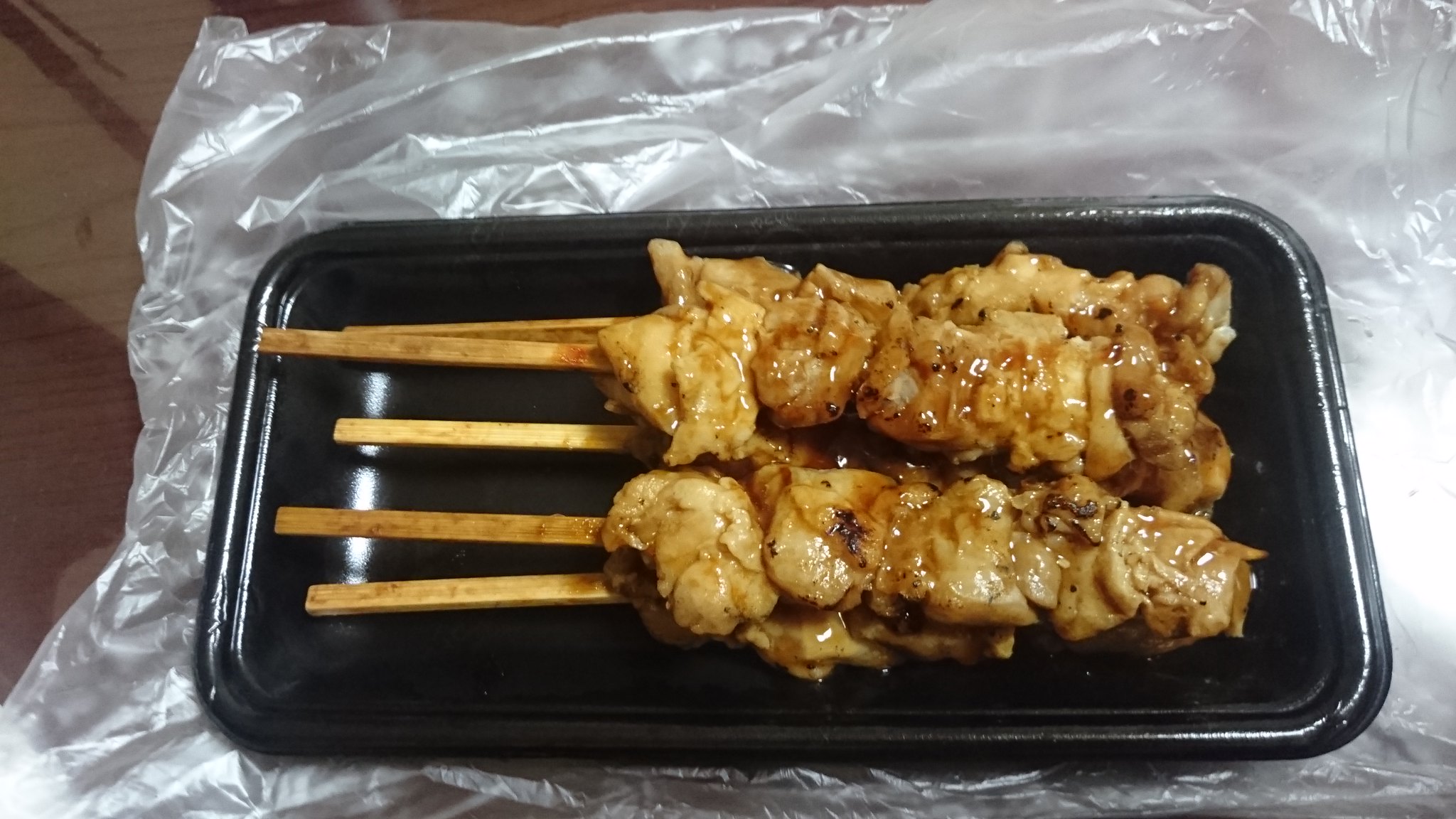In this color photograph, displayed in landscape format, we see a black rectangular tray containing five long, narrow skewers of succulent yakitori, a type of grilled Japanese chicken on sticks. The yakitori appears juicy and glistening, possibly due to a soy-based sauce, and is positioned on the right half of each skewer, leaving the wooden sticks visible on the left. Each skewer holds several browned, glossy pieces of chicken tightly packed together. The tray, reminiscent of takeout packaging, sits atop a clear plastic sheet on a wooden surface with light brown and white streaks running vertically. Additionally, a plastic bag, likely the original packaging for the skewers, is also present on the tray.